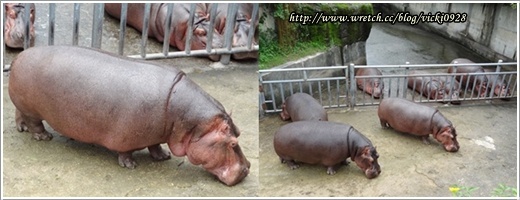The image consists of two side-by-side photographs, likely sourced from a book or magazine, depicting hippopotamuses in a zoo environment. The left photo is a close-up of a single large hippo with a brownish-pink hue, standing near a sturdy metal fence. The right photo is a wider shot of the same scene, showing a total of eight hippos. The enclosure has a concrete ground with three hippos in the foreground and five hippos on the other side of a water area, separated by the metal fence. Some of the hippos appear to be sniffing the ground. In both images, the hippos' enclosure is visibly a well-defined space within a zoo, with water visible in the background. The page also includes a small, unreadable website link in one corner.